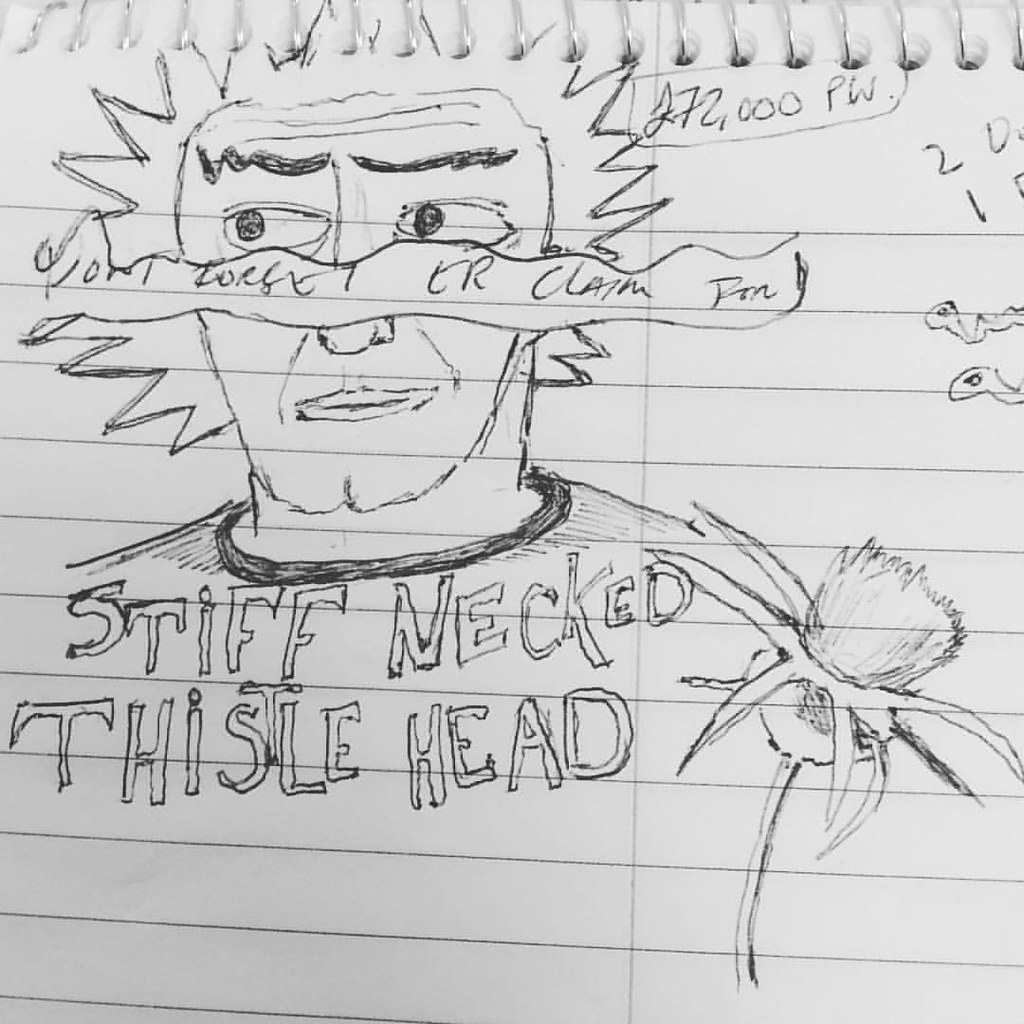This is a detailed pencil and pen drawing on a sheet of lined white paper, characterized by faint black horizontal lines and a single vertical line down the center. The paper features silver wire coils at the top, indicating it comes from a spiral notebook. The drawing depicts a man from the neck up, with a square, yet slightly rounded jawline, spiky hair resembling little triangles, squiggly eyebrows, and lines etched into his forehead. A squiggly rectangle with illegible text stretches across his face.

The man is wearing a shirt with a dark collar, though only faint shoulder lines are visible. Above the man, at the top of the page, the text "272,000 PW" is written. Below the drawing, bold block letters proclaim "stiff-necked thistlehead." Adjacent to this text, there is a detailed drawing of a thistle, complete with a stem, pointed petals, and leaves near the top. Additionally, a couple of snakes are depicted slithering in from the sides of the page, adding a distinct touch to the composition. The entire piece is rendered in black ink, with detailed attention to the finer elements, such as the spikes in the hair and the intricacy of the thistle.